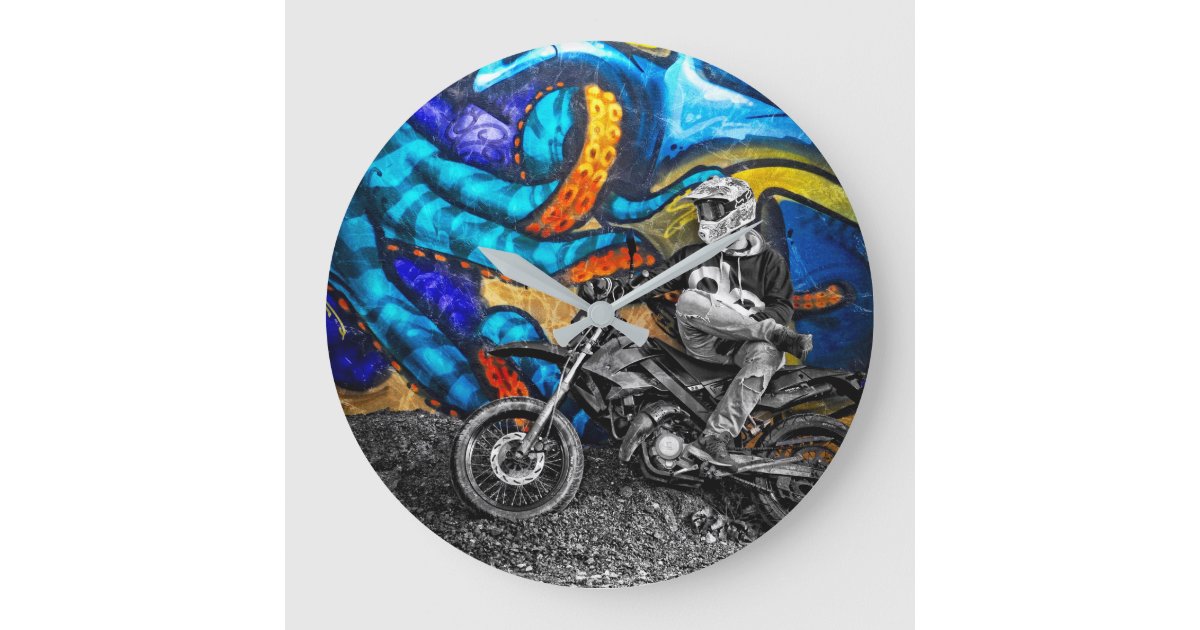The image depicts a clock with a round face set in a gray square background that gives the appearance of a metallic shield or button. In the center of the clock face is a striking photograph of a man sitting on a silvery grey motorcycle, which leans against a wall adorned with an exuberantly colorful mural of an octopus. The man, wearing a white motorcycle helmet, a black and white sweater, white pants, and black shoes, sits on the motorcycle with his legs crossed. Notably, both the man and his motorcycle are depicted in black and white, contrasting sharply with the vivid mural behind them. The clock has silver hands indicating it is 10:10, but lacks numerical markers, making it purely ornamental. The ground beneath the motorcycle is depicted as grey gravel, blending flawlessly into the monochromatic theme of the man and his machine. The overall effect is a captivating juxtaposition of grayscale subjects against a rainbow-hued backdrop, all within the functional yet enigmatic design of the clock.